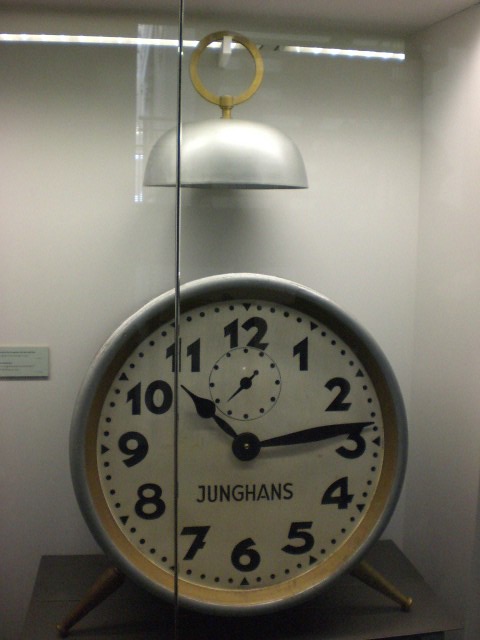The image features a large, antique alarm clock encased behind glass, reminiscent of a museum exhibit, suggesting its historical or cultural significance. The clock, while grand in size, emulates the design of a traditional bedside wind-up alarm clock. It appears to be divided into two distinct sections: the lower part, resembling an everyday alarm clock with a standard clock face, and the upper part, which is strangely detached. The upper section includes a silver cap and a golden ring, synonymous with the bells typically found on vintage alarm clocks. The clock face bears the name "Jungens," a term that likely reflects either the manufacturer or a specific model, though its exact origin remains unclear. This presentation hints at the clock’s potential importance, whether historical, technical, or decorative, meriting its sequestered display.